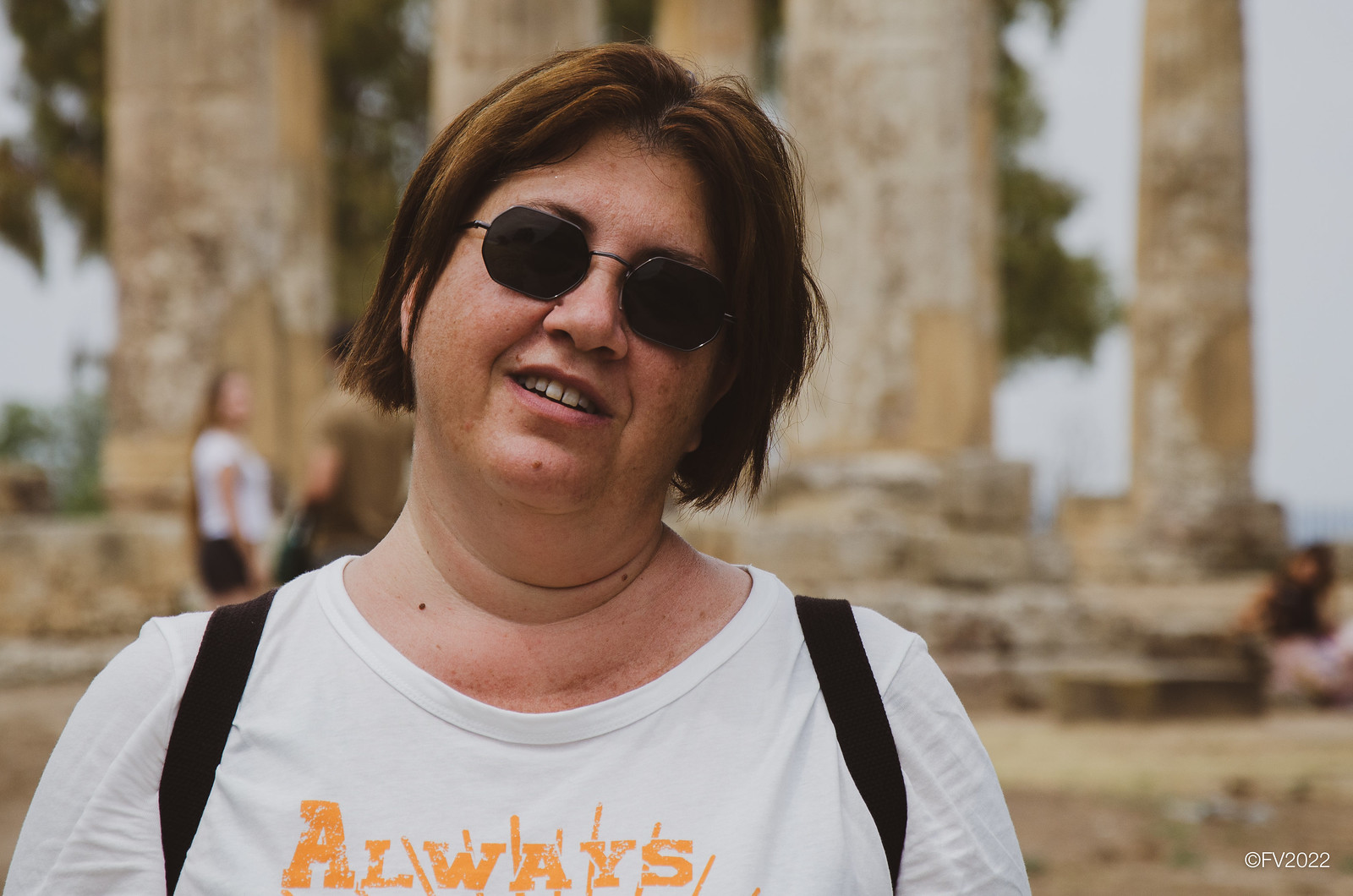The photograph features a woman from the chest up, standing in the foreground. She wears a white graphic t-shirt with partially visible orange letters spelling "A-L-W-A-Y-S," intersected by multiple lines. Two black backpack straps are visible over her shoulders, although the backpack itself isn't seen. She sports black-rimmed, black-lens sunglasses with an octagonal shape, lending a distinctive look. Her brown hair, which has a slight reddish tint, falls just below her ears, and her head is slightly cocked to the right. Noteworthy facial details include a few moles—one on her chin, one on her neck, and one on her nose, as well as a slight gap between her front teeth.

In the background, the image reveals the ruins of an ancient Mediterranean structure, characterized by various deteriorating marble pillars. This historical setting suggests a location rich in cultural heritage, possibly Greek or Roman. The entire scene is subtly marked by a watermark in the bottom right corner, reading "copyright FFVS 2022," indicating the image's ownership and date.